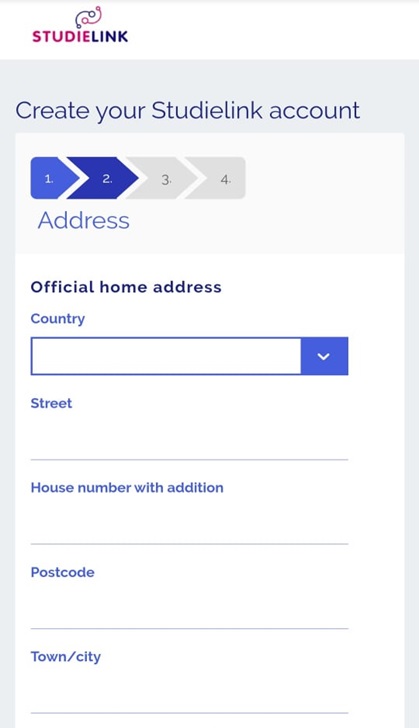The image is a mobile screenshot displaying a webpage for setting up a Studielink account. The background of the page is predominantly white, divided by a thin gray horizontal line running from left to right at the top. On the upper left corner, "Studielink" is written, with "study" in purple and "link" in black. Adjacent to the text is a logo featuring two curved lines—one black and one purple, each ending in small circles.

Beneath this header, there is a gray vertical box containing the text "Create your Studielink account" in dark font. Inside this, there's a thinner, lighter gray box with the word "Notes" in blue. A flowchart depicted with a sequence of numbers—1 and 2 in blue, and a continuation to 4—illustrate steps in the account creation process.

Further down, there's a white input box titled "Official home address" in black. Below this, fields for entering personal information are laid out, beginning with a drop-down menu for selecting a "Country," accompanied by a blank blue button. Following this are input fields labeled "Street," "House number with addition," "Postcode," and "Town/City," each with lines for the user to provide their details.